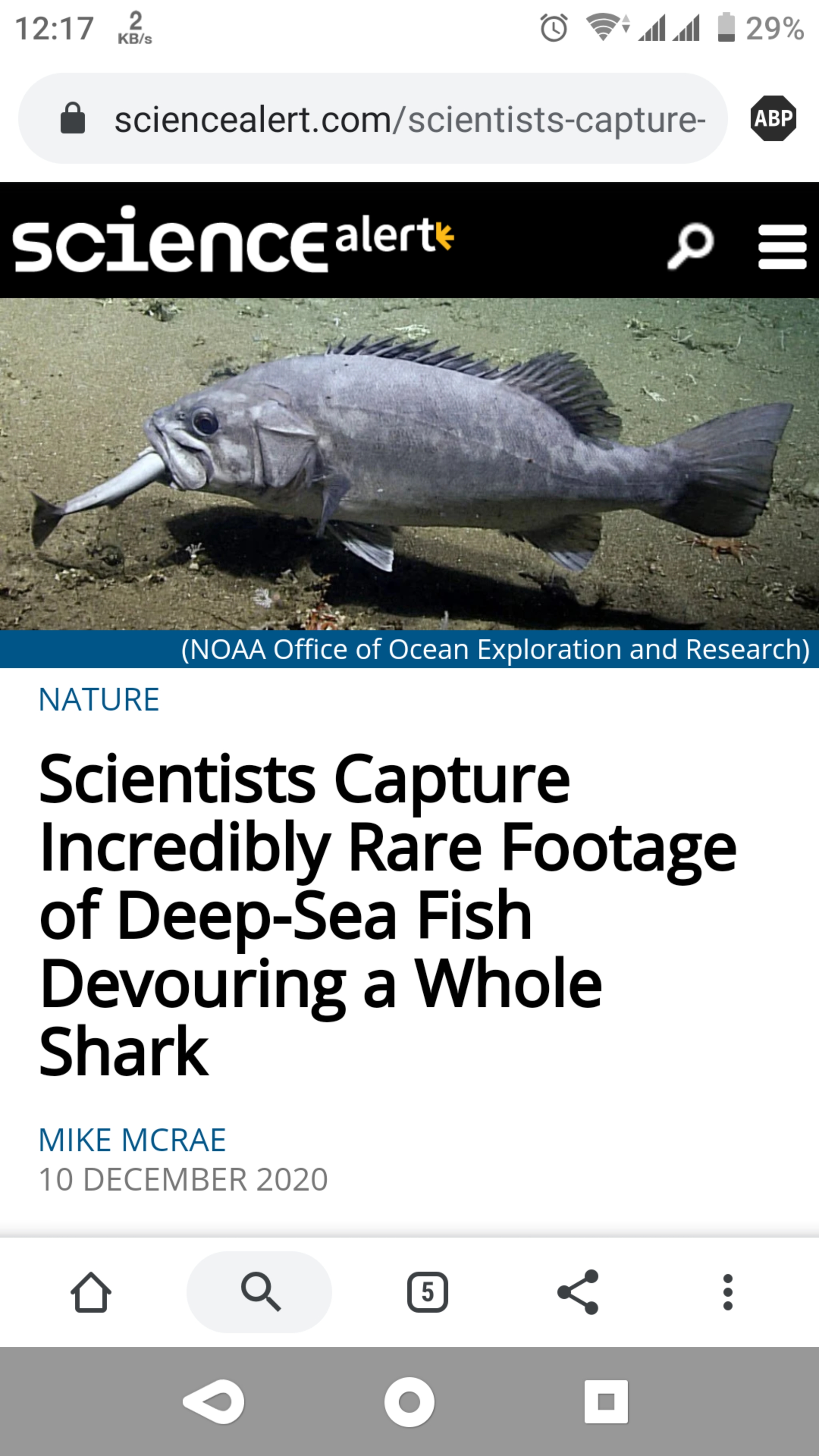This mobile phone screenshot captures a webpage on ScienceAlert.com, displayed with a 29% battery life visible in the top right corner and the time shown as 12:17 in the top left corner. The URL of the website appears at the top of the screen. 

Prominently featured in the center is an image of a gray-colored fish swallowing another fish, with the tail of the prey fish protruding from its mouth. The webpage title, "ScienceAlert," is clearly visible beneath the URL. Directly under the image, the article title reads, "Scientists Capture Incredibly Rare Footage of Deep-Sea Fish Devouring a Whole Shark," authored by Mark McRae and published on December 10, 2020. The webpage has a clean, all-white background. 

At the bottom of the screen, the phone's navigation keys are displayed, including the back button, the center menu key, and the square-shaped recent apps button.